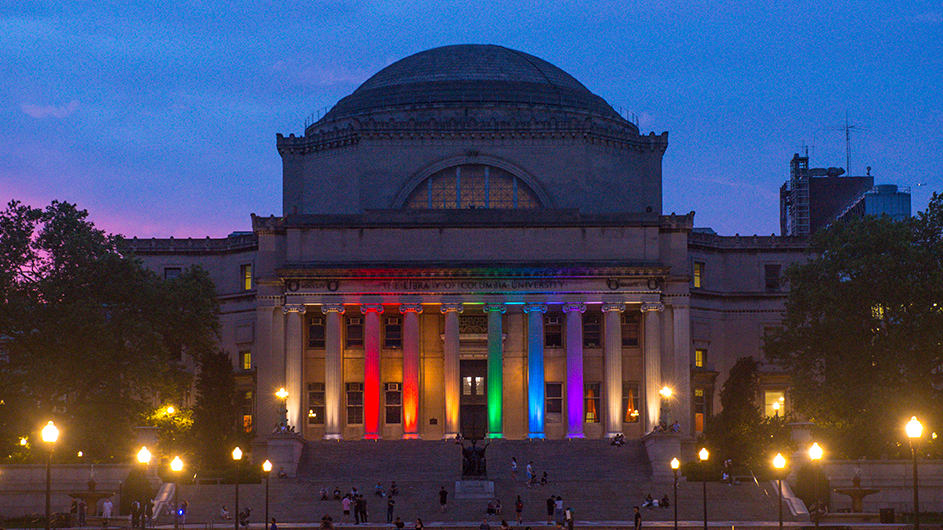The image depicts a large, rectangular horizontal government building adorned with lighted pillars in rainbow colors, likely in support of Gay Pride Week. The building's front features a long flight of stairs leading up to an entrance framed by columns illuminated from red to violet. Above the pillars, a grand dome with an arched window presides over the scene. As dusk sets in, the sky transitions from blue to purple hues, especially noticeable in the left corner, while street lights and potential car headlights hint at the evening's progression. Large trees with full foliage flank either side of the building's entrance, and a few people are visible ascending the stairs. This celebratory lighting, combined with the building's architectural details, suggests a significant and historic structure, reminiscent of but not definitively identified as the U.S. Capitol.